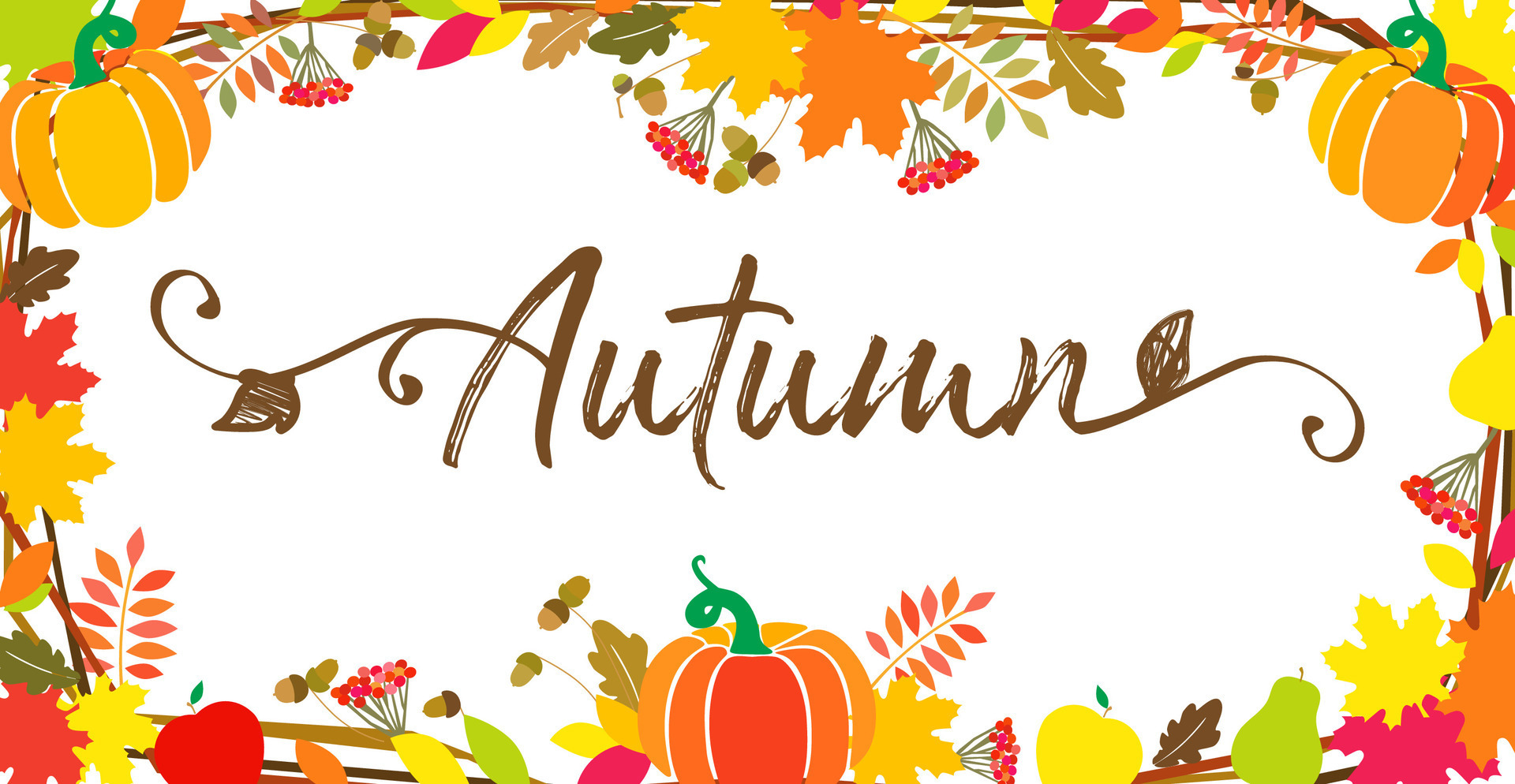This image is a rectangular art print with a white background and a vibrant depiction of autumnal themes. In the center, the word "Autumn" is elegantly written in brown cursive, featuring flourishing curves extending from both the capital 'A' and the final 'N'. These curves intertwine with small brown leaves, enhancing the festive feel. Surrounding this text, a rich frame showcases an array of fall-themed elements. In the upper corners and the bottom center are pumpkins, each section displaying varying shades of orange and yellow, complemented by bright green, swirling stems. The border of the artwork is adorned with a mix of fall staples: multicolored maple leaves in hues of orange, brown, yellow, and bright pink, green pears, red and golden apples, twigs, and both red and pink berries. Accents of acorns and brown sticks contribute to the intricate, colorful frame that encapsulates the essence of the autumn season.